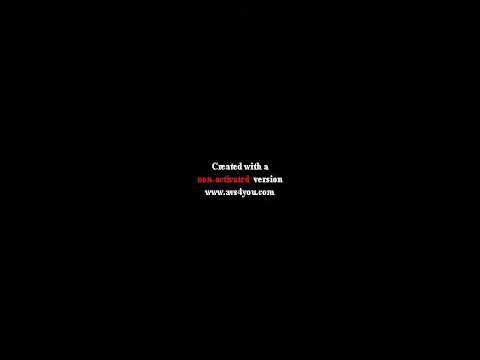The image features a very simple and low-quality screenshot with a predominantly black background. At the center, there are three lines of blurry and almost unreadable text. The text states "created with a non-activated version," with "created with a" and "version" in white and "non-activated" in deep red. Beneath this message is a URL in white text, which is difficult to fully discern apart from the "www" at the beginning and the ".com" at the end. The overall appearance is that of a basic, almost postcard-like image, alerting viewers of its non-activated status with minimal detail on a stark black backdrop.